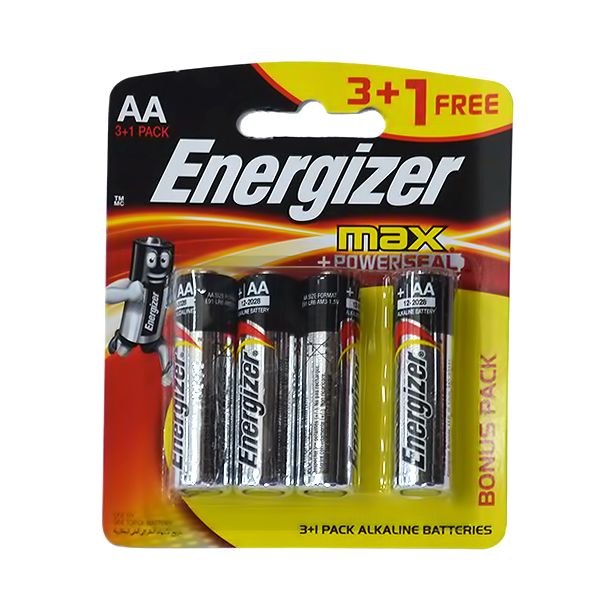This image showcases an Energizer pack of AA batteries, prominently featuring the brand name "Energizer" in large, white letters on the package. Positioned in the top right corner is a yellow section with red fonts and numbers stating "3 + 1 Free." The package contains four batteries arranged with a noticeable gap between the third and fourth battery, indicating the free battery. Each battery has a predominantly silver cylindrical body with the top quarter in black. The black section bears the label "AA" in white letters, followed by a white bar with additional numbers and lettering, including the text "alkaline battery."

At the bottom of the package, the phrase "3 + 1 Pack Alkaline Batteries" is printed in black. On the right-hand side, "Bonus Pack" is typed in red letters. Each battery itself bears the "Energizer" branding in black, accompanied by distinctive red and yellow wisp designs. 

To the left of the batteries on the packaging, there is an animated character resembling a battery, complete with expressive eyes and a mouth. This battery man wears shorts and appears in a dynamic running pose, with his right leg pulled back and up, left leg extended forward, and right arm raised in a fist. The background of the package consists of a black section behind the "Energizer" text, with the area behind the batteries themselves mostly filled with yellow and accents of wavy lines.